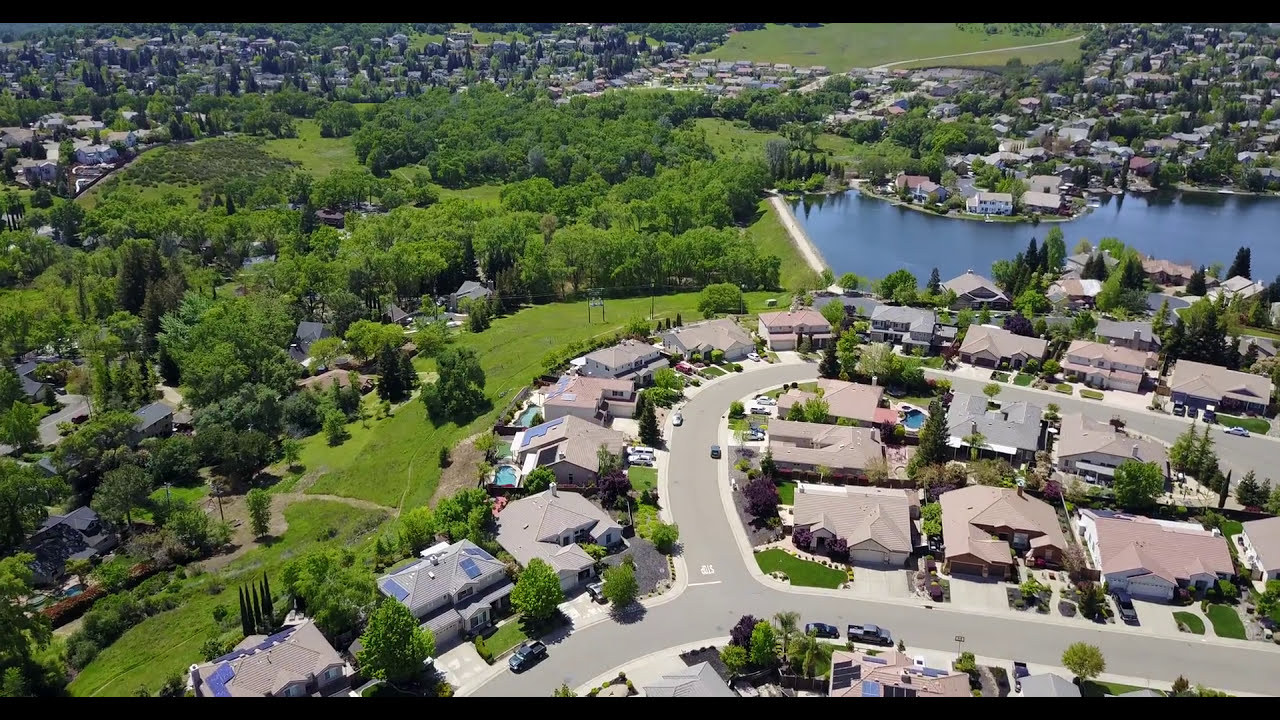This aerial photograph, captured from approximately 100 feet above, showcases a typical American suburban neighborhood bathed in daylight. The image teems with details of single-family homes, each occupying small plots of land but relatively close to one another. The houses, averaging around 1,500 square feet, boast features such as solar panels and backyard pools. 

The neighborhood streets are visibly clean and nearly empty, with most cars parked in driveways. The road network is intricate, with a prominent street visible that branches off into three directions near the bottom edge of the image. Throughout the scene, lush greenery is abundant; trees and expanses of grass provide a verdant backdrop to the residences.

In the lower right portion of the frame, the suburbs extend densely, while further to the upper right, a serene blue pond punctuates the landscape, flanked by a continuous stretch of houses. A potential park area, marked by its grassy terrain and clusters of trees, lies to the left. The horizon reveals more suburban sprawl, with a large body of water further demarcating the right side of the image. The scene is framed with a thin black header and footer, completing this vivid representation of suburban life.